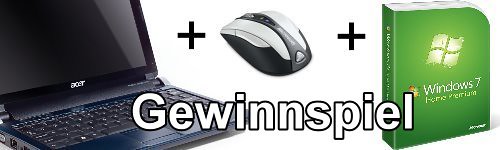This is an advertisement showcasing a technology bundle. The word "Gewinnspiel," meaning "competition" or "game" in German, is prominently displayed in bold white text outlined in black across the lower center of the image. The background is entirely white, creating a clean and minimalist aesthetic.

On the left side of the image, there is an open Acer laptop with a black screen, partially displaying the keyboard. In the center of the image, there is a black and white computer mouse. To the right, there is a green package showing the Windows 7 operating system, with the Windows logo slightly visible and adding a touch of color.

The layout of the items follows a sequence: the laptop, followed by a plus sign, then the mouse, another plus sign, and finally the Windows 7 package, all laid out against the white background. The only colors present in the image are black, white, green, and a small hint of color within the Windows logo.